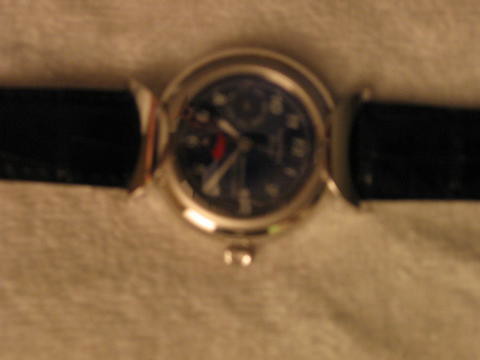An indoor, color photograph captures a watch with a black band, possibly leather or plastic, laid horizontally against a light tan, possibly carpeted, background. The image is blurry and out of focus, making fine details challenging to discern. The watch features a round gold body with a black face, adorned with white numbers and gold-colored hands, pointing to 1:50. A small dash of red is visible on the face, adding a subtle detail. The crown or knob for setting the time is located at the bottom center of the watch face. The watch straps are thin, rectangular, and black, emerging from crescent-shaped attachments on both ends of the watch frame. Light reflections are present on the lower left side of the gold case, highlighting its polished surface. Overall, despite the blurred quality of the image, the watch appears to be in very good condition.